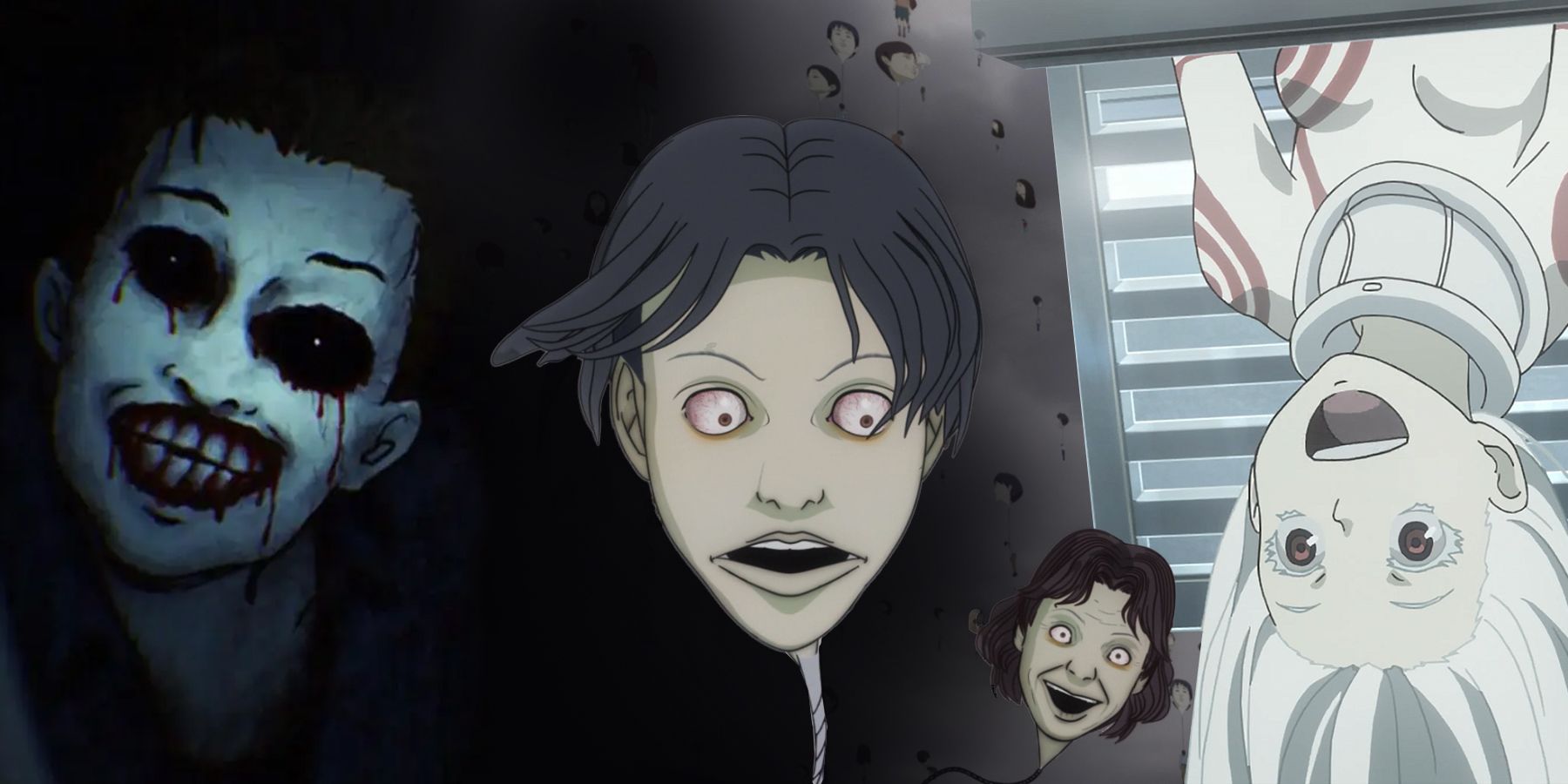The image is a highly detailed, anime-style illustration with a distinct horror or gothic theme, presented in landscape orientation. On the left-hand side, there is a menacing zombie-like figure with a white face, black eyes, and large teeth, with blood dripping from its eyes and mouth, creating a sinister smile. Moving towards the center, there are two heads that resemble balloons, each attached to a cord extending out of the frame. These heads have bulging, bloodshot eyes and open mouths, conveying a look of shock or surprise. Both have brownish hair. On the right side, upside-down and appearing to emerge from a doorway or window with light behind her, is a female figure with wide eyes and an open mouth. She has white hair and is adorned in a sci-fi-inspired white bodysuit decorated with red, target-shaped markings on her shoulders and breasts. The overall composition of the image combines elements of bright and dark tones, enhancing its eerie and unsettling atmosphere.